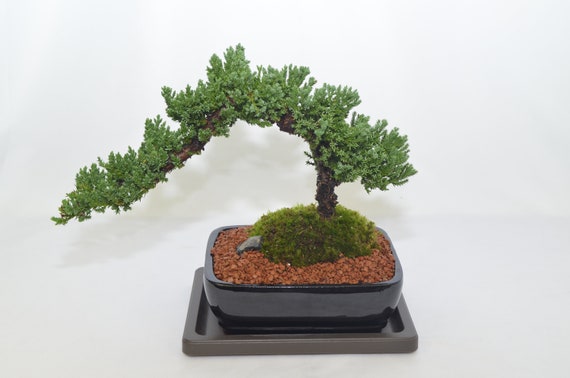This image showcases a meticulously manicured bonsai tree set against a stark white background, highlighting its intricate details. The bonsai is planted in a rectangular, black ceramic dish, slightly shiny with curved edges, which sits atop a thin, flat brown tray that appears to catch excess water. The base of the bonsai tree is surrounded by small reddish-brown rocks and a prominent ball of green moss, creating a miniature hill-like effect. The trunk ascends gracefully before curving to the left, where a long, elegant branch stretches across nearly the entire left side of the image. This branch and others are adorned with short, dark green evergreen needles, possibly indicating a juniper variety. The tree appears well-pruned and carefully looked after, casting a subtle shadow on the white backdrop.